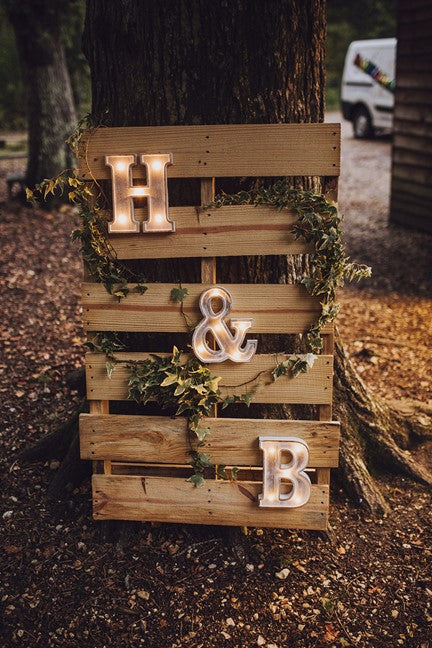This image captures a rustic outdoor wedding scene. At the center is a large, old tree, against which a light-colored wooden pallet leans. Interwoven with ivy, the pallet features three semi-transparent, white illuminated letters: 'H,' an ampersand '&,' and 'B,' all lit from within by warm yellow LEDs. The letters are arranged diagonally from the top left to the bottom right of the pallet. The surrounding ground is a mix of dirt, fallen leaves, and scattered rocks and sticks, suggesting a fall setting. In the background, another tree stands to the left, while to the right, a gravel parking area is visible. A white van is parked in front of a house with wooden siding, which also partially appears in the frame. The overall ambiance suggests a rural, intimate wedding celebration.